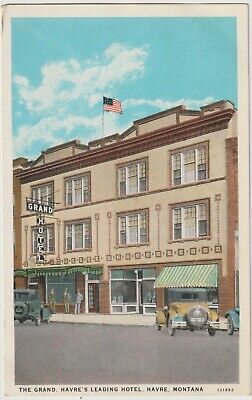The image, likely a hand-painted scene on a white backdrop, depicts a nostalgic downtown setting from the 1940s. Dominating the foreground is the facade of a three-story building labeled "Grand Hotel." The hotel's exterior is constructed from tan, stone-like material, accented with darker brown squares above the first floor, and features a total of eight windows divided into two sections. A green striped awning extends from the building's entrance, providing a welcoming touch.

Parked in front of the hotel on the street are two vintage cars, one greenish and one gray, both embodying the classic boxy design with skinny tires and rear-mounted spare wheels typical of the era. Above the hotel's entrance, a sign reads "Grand" horizontally with "Hotel" vertically beneath it in white letters on a black background. Atop this historic structure, an American flag waves proudly against a blue sky dotted with wispy clouds.

Beneath the hotel's name, the inscription reads "The Grand, Havares Leading Hotel, Havare, Montana," further grounding the image in a specific place and time.